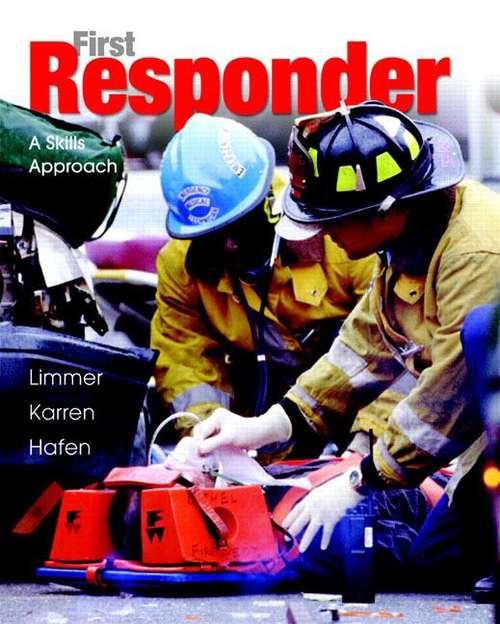The image is a detailed cover for a book titled "First Responder: A Skills Approach." At the top, the title is prominently displayed with "First" in gray text and "Responder" in large red text. Below the title, in smaller white text, is the subtitle, "A Skills Approach." The middle left of the cover lists the authors' names: Limmer, Karin, and Hafen in white text.

The cover features an intense and realistic scene with two first responders, possibly paramedics or firefighters, who are kneeling on the ground attending to an injured individual. One responder is a white man wearing a black helmet with a neon green stripe, and the other is a black man wearing a turquoise blue helmet. Both responders are clad in yellow jackets with silver reflective bands. The responders' faces are not clearly visible as they are looking down and focused on administering aid.

The injured person lies on a stretcher with red head blocks for neck stabilization, and the responder on the right is seen wearing gloves and holding an oxygen mask over the victim's face. The scene suggests an emergency, likely a car crash, highlighting the critical and skillful interventions of the first responders in action.